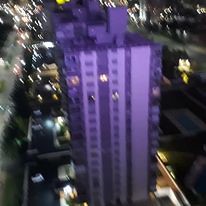The image is a square, low-resolution, nighttime color photograph taken from a high angle, possibly from a building or a drone. The central focus is a tall, 30-40 story high-rise tower block that dominates the frame, appearing entirely illuminated in a distinctive mauve or purple hue. The photograph presents a blurred effect, likely due to a slow shutter speed and slight movement during capture. Surrounding the prominent building are a parking lot and various streetlights and vehicle headlights, creating streaks of light as they extend diagonally to the right, indicating the bustling activity of a populated area. Additional details reveal highways and numerous properties around the base of the tower, emphasizing the urban setting of the shot.